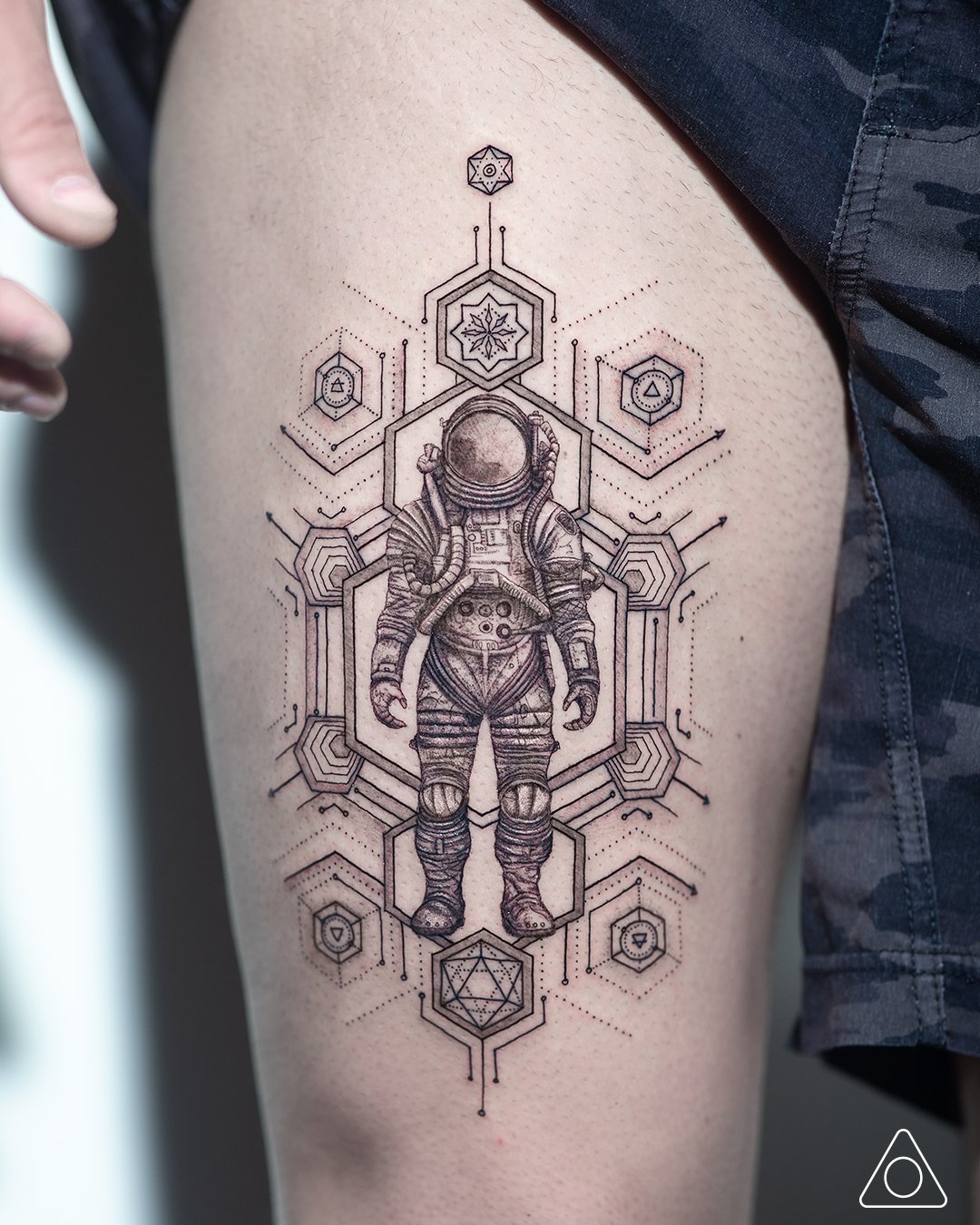This image features a highly detailed black and white tattoo on a person's upper thigh, spanning from just above the knee to the upper thigh. The individual has pale skin and is wearing black and gray camouflage shorts, which are partially rolled up to showcase the tattoo. The tattoo depicts an astronaut standing face-on to the viewer, dressed in a futuristic spacesuit with meticulous line art involving rows of dots and extensive shading. Surrounding the astronaut are various interconnected geometric patterns, primarily hexagons, but also including other shapes like triangles and a dodecahedron. These patterns feature intricate designs within them and are connected by fine lines and dots, giving the tattoo a complex, mandala-like appearance. In the lower right corner of the tattoo, there's a logo consisting of an equilateral triangle with rounded corners, featuring a circle at its center. The person's hand, visible at the upper left corner of the image, appears to be pulling up the shorts to better display the tattoo. The background is white, accentuating the intricate black linework of the tattoo.